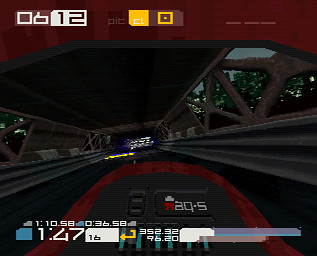The image shows a dimly lit first-person perspective from a racing video game, reminiscent of older consoles like the Sega Genesis or Nintendo 64. The screen is almost square, presenting a constrained, close-up view. We appear to be inside a vehicle, potentially a car or motorcycle, with a brown dashboard accented by a darker brick-red outline. A heads-up display (HUD) is visible, showing various numbers and indicators: an 80.5, 71 in red, and an elapsed time of 147, suggesting a race scenario. The top left corner displays the numbers 6 and 12, likely indicating a position, such as being in 6th place. The scene depicts the vehicle racing along a covered or lower deck of a bridge at night, supported by metal girders forming X and vertical bar patterns on both sides. Through the sides of the structure, a nighttime cityscape is faintly visible, adding depth to the gaming environment.